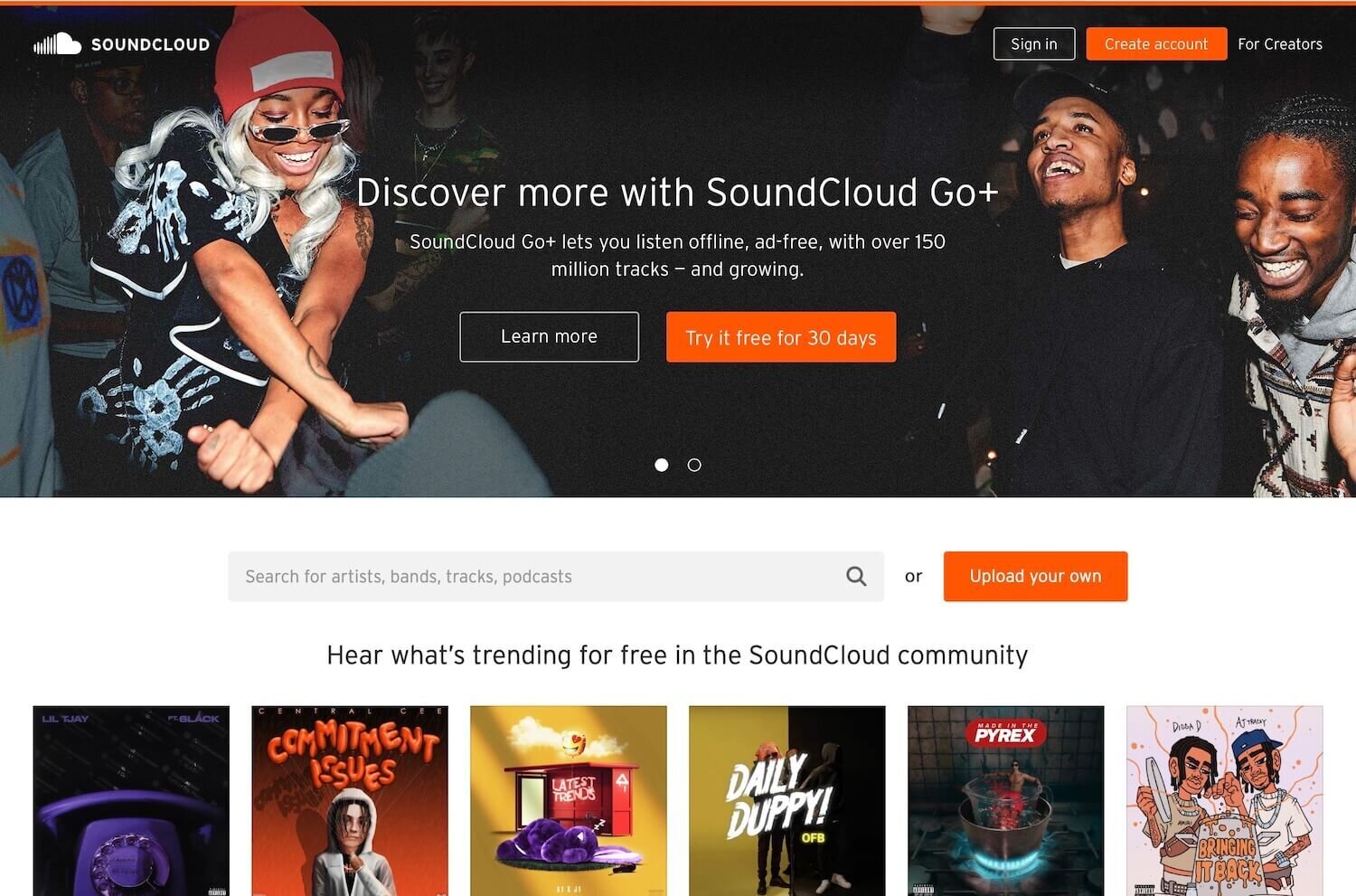Screenshot of SoundCloud Homepage (Not Logged In):

The screenshot captures the SoundCloud homepage for users who are not logged in. In the top left corner, the iconic SoundCloud logo is positioned with the cloud icon to the left. The main section features a dark-themed promotional banner for SoundCloud Go+, encouraging users to "Discover more with SoundCloud Go+" which offers benefits like offline listening, an ad-free experience, and access to over 150 million tracks. Below this message, there are two prominent buttons: a grey "Learn More" button and an orange "Try it free for 30 days" button, inviting users to explore the service.

In the top right corner, several user navigation options are visible: a "Sign In" button, an orange "Create Account" button, and a "For Creators" link. Positioned beneath this header is a search bar where users can look up artists, bands, tracks, and podcasts. Next to the search bar is an orange button labeled "Upload Your Own," encouraging creators to add their content to the platform.

The lower section of the page highlights trending tracks from the SoundCloud community, titled "Here's what's trending for free in the SoundCloud community." This section showcases six album covers, each with titles and featured artists including:
- "Little TJ featuring Six Flack"
- "Central Sea's Commitment Issues"
- "Latest Trends"
- "Daily Duppy"
- OFB's "Made in the Pyrex"
- "Bring It Back," by Dissidy and AJ Tracy

This snapshot provides a comprehensive view of the SoundCloud homepage, highlighting its main features and user navigation options.